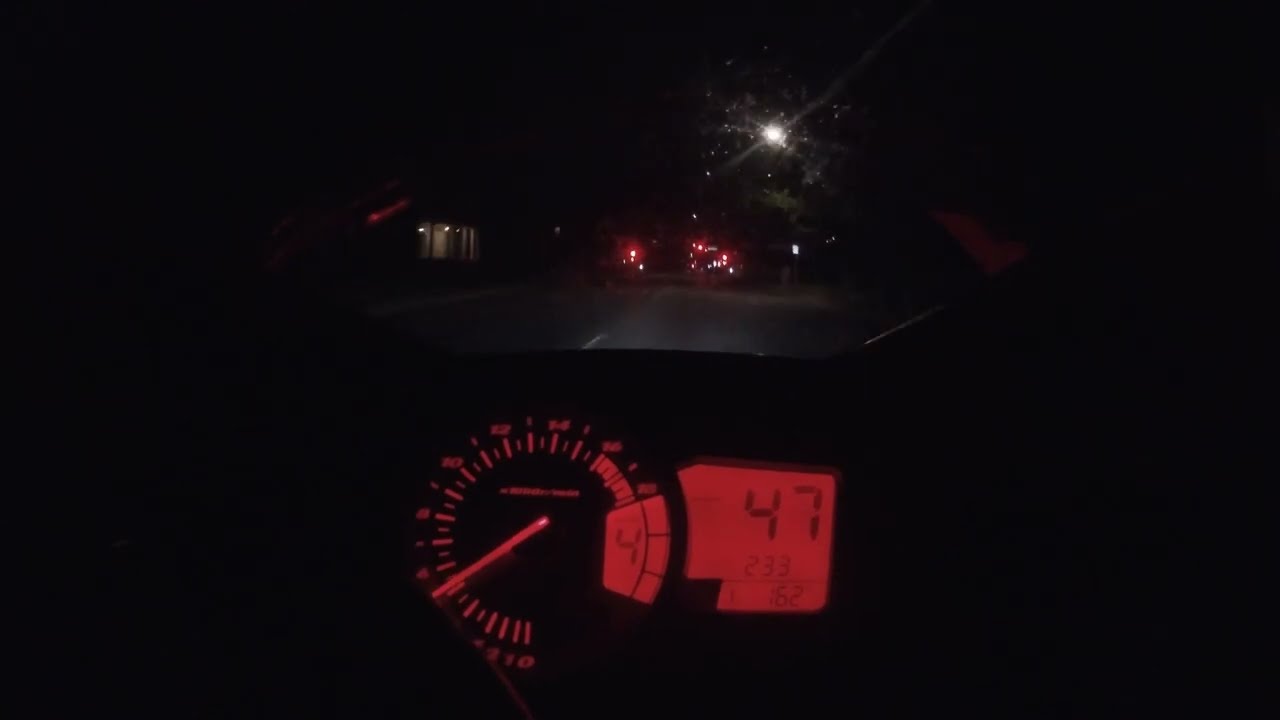This nighttime photograph is captured from inside a moving vehicle, showing the driver's perspective. The scene outside the car is very dark, with the only visible features being a structure with lit windows to the left of the road and a distant streetlight. The main focus inside the vehicle is a well-lit speedometer with red illumination, indicating the car is traveling at 47 miles per hour. This speedometer also displays additional numbers; notably, the number 233 below the speed and the number 4 on the left. Farther ahead on the road, red traffic lights add to the sparse lighting. The entire interior of the car, except for the illuminated speedometer, remains largely in darkness, with a hint of an object possibly sitting on the dashboard. There are no other vehicles visible on the presumably empty road.